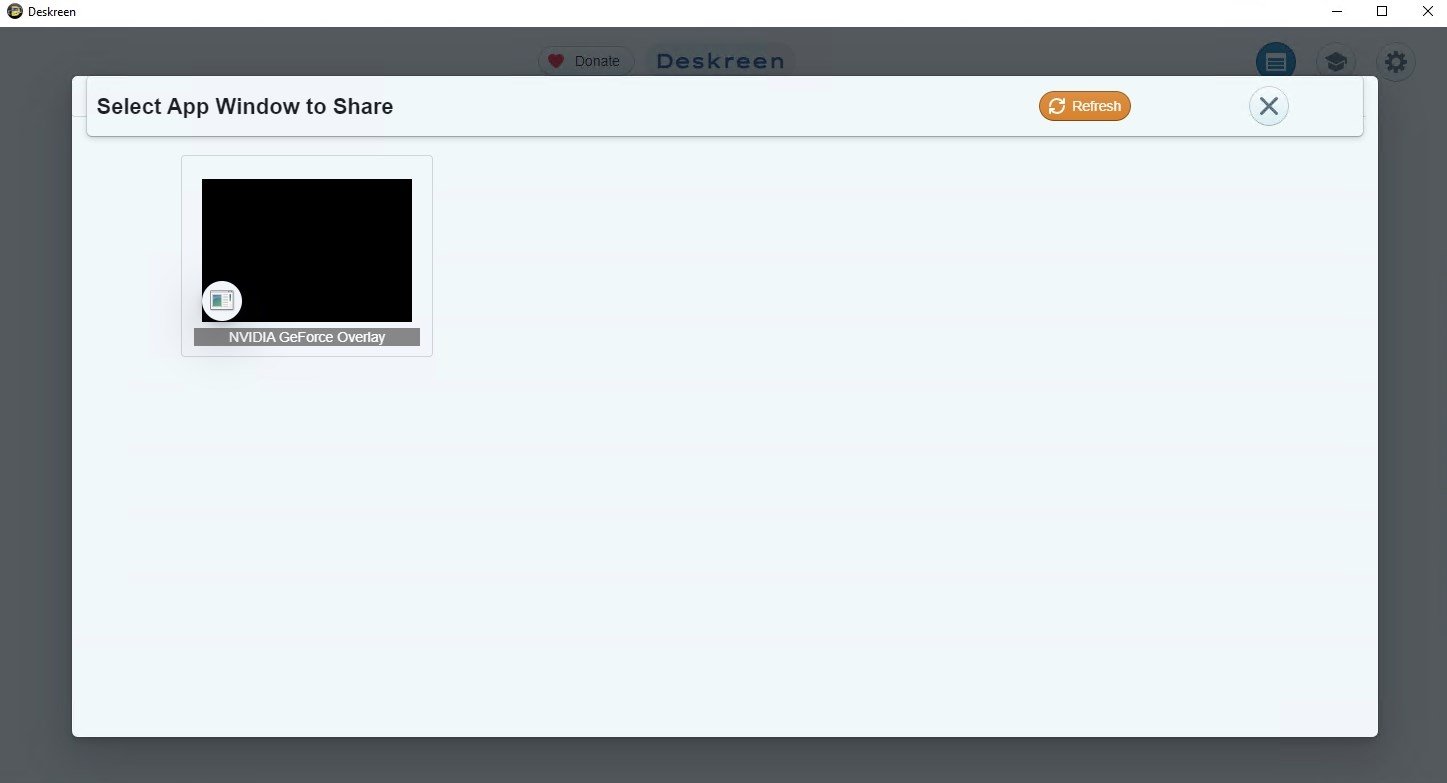The image is a screenshot displaying a software application called Deskreen. This application window has a white background with the Deskreen logo positioned in the upper left corner, next to the word "Deskreen" in black text. In the upper right corner of the window, there are the standard window control buttons: minimize, maximize, and close (represented by an "X").

The main content of the screenshot shows the application window in a grayed-out state, indicating it is not currently active. Overlaying this window is a light gray pop-up dialog box. At the top of this pop-up, the header reads "Select app window to share," accompanied by an orange refresh button with white text and an "X" button to close the dialog.

Below this header, the pop-up features an outlined black square that contains an inset image of a Windows logo, suggesting a specific application or window available for sharing. Underneath this image, there is a gray box with white text that reads "NVIDIA GeForce Overlay."

In the background, behind the pop-up, the Deskreen application window shows additional interface elements, despite being grayed out. At the top of this window, there is a "Donate" button with a heart icon next to it, "Deskreen" in the middle, and on the far right, there are three icons: a window icon, a graduation cap outline, and a settings gear icon.